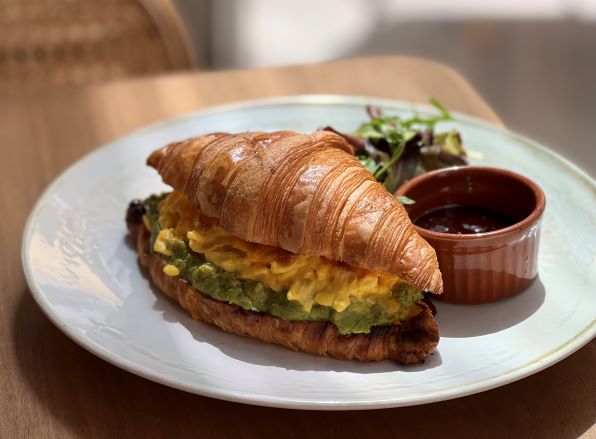This photograph showcases a detailed still-life composition featuring a croissant sandwich and accompanying elements. The sandwich itself is made from a golden-brown toasted croissant, which may be slightly darker on its bottom half. The sandwich filling includes a layer of green avocado spread at the base, topped with a yellowish, clumpy mixture that could potentially be scrambled eggs or an egg salad. The sandwich is placed on a pristine white plate, which rests on a wooden table. To the right of the sandwich, a small, brown ramekin contains a reddish-brown sauce or dressing. Behind the main focus of the croissant sandwich, there's a small, fresh salad that appears to include mixed greens, possibly arugula, rather than just iceberg or romaine lettuce. The background features a hint of a wooden chair that is slightly blurred, along with a gradient blur from white to dark grey. The image captures the colors vividly, with green, yellow, brown, and touches of red, all set against the natural tones of the wooden table and the neutral background.